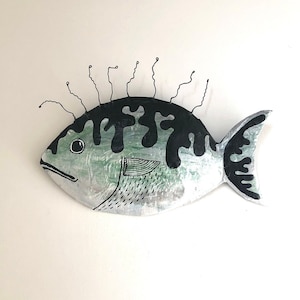The image depicts a detailed model of a medium-sized fish mounted on a blank, beige-colored wall. The fish has a rounded, plump body with a distinctive coloration scheme: its top is marked with irregular black splatters that drip down like melting ice cream, blending into a green midsection and a white belly. The black splatter patterns are also observed on its dorsal and tail fins. The fish has a shiny, silver, and scaly texture, with a round black eye and simple, straight black lines illustrating its mouth, which gives it a somewhat nervous expression. There are approximately eight antenna-like wires protruding from the top of its body, bending and curving in various directions, adding a whimsical touch. Additionally, a small fin is drawn on its side, accompanied by penciled-in gray scales to enhance the illusion of texture.